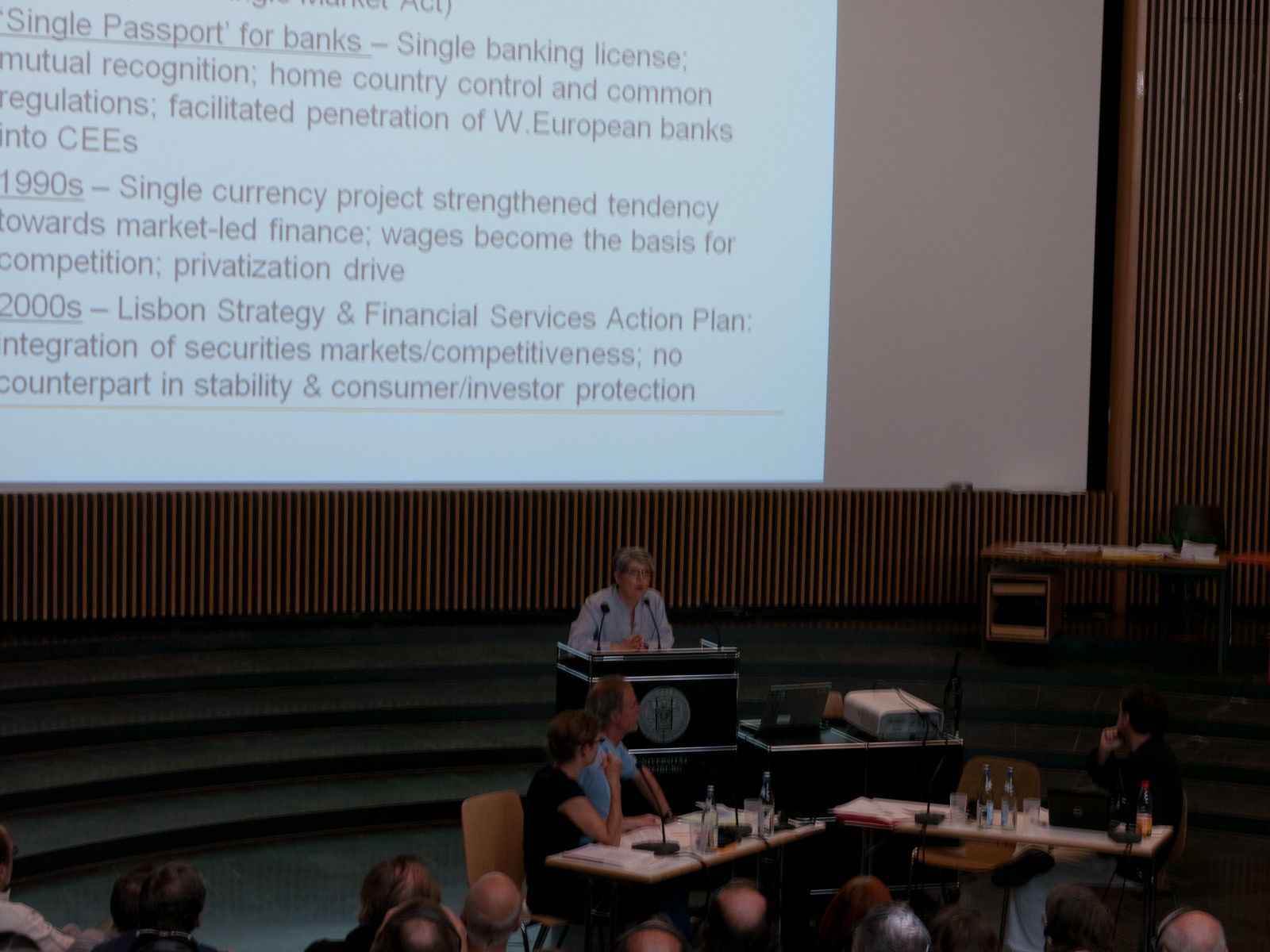The image depicts a detailed scene inside an auditorium where a financial presentation is taking place. An older woman with gray hair, dressed in a light blue long-sleeved shirt, stands at a black podium with a logo on it, presenting to an audience. The large screen behind her displays a PowerPoint slide outlining various financial topics such as single passport for banks, mutual recognition, and the Lisbon strategy. Seated in the foreground are two triangularly arranged tables laden with white papers and water bottles. The left table shows two people turned to their right, while the right table has one person looking back at the speaker. The audience comprises around 8-10 mostly middle-aged individuals, some balding, attentively listening and looking at the presenter and the screen. The setup strongly suggests that this meeting is intended for investors or financial professionals, underscoring the themes of market integration and finance.